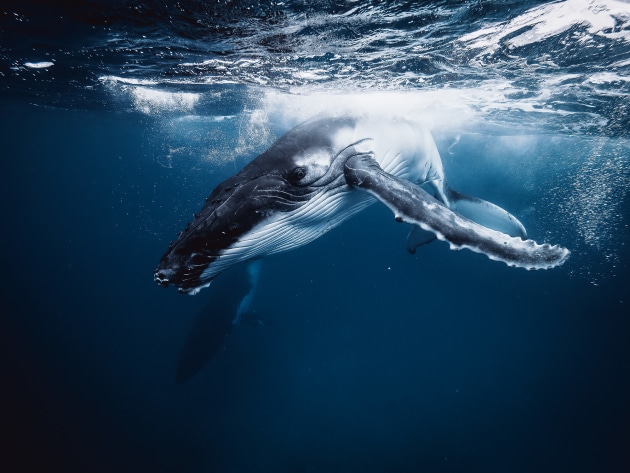This captivating image showcases a majestic adult humpback whale near the ocean's surface, captured in a serene underwater scene. The whale, having just breached the water to get air, is now diving back down with its fins extended, showcasing its impressive white-striped underbelly and dark-blue to black top speckled with barnacles near its mouth. The water is exceptionally clear, allowing sunlight to illuminate the whale and the few bubbles floating upward from its recent surfacing. The whale is positioned towards the surface, with sunlight reflecting through the water, highlighting its powerful form and the serene ocean environment. In the backdrop, a faint shadow suggests the presence of another whale deep below, adding depth to this stunning marine tableau.